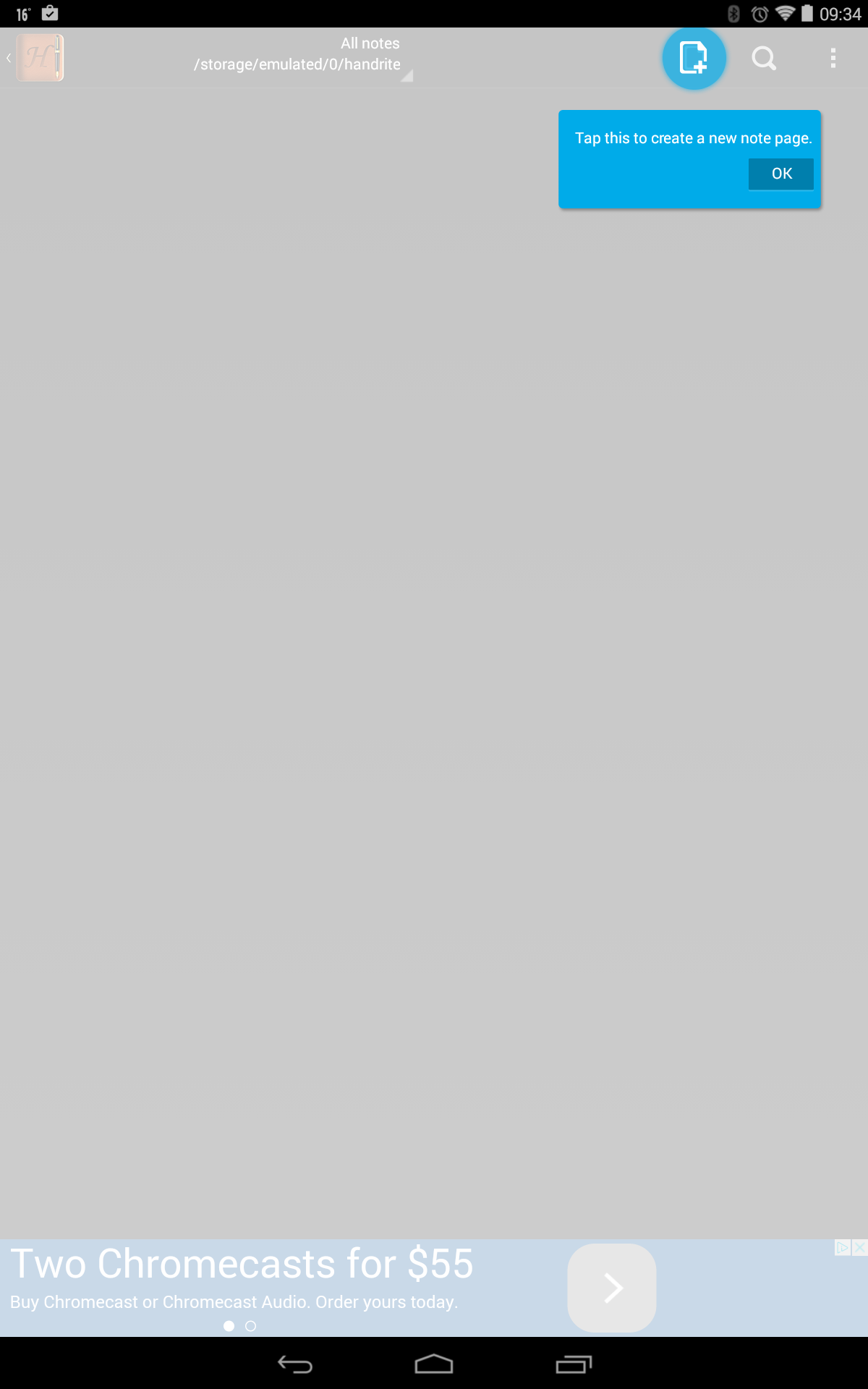This screenshot from a smartphone showcases a user interface with several key elements. The background is a uniform grey color. At the top of the screen is a highlighted icon for adding a new note, marked by a blue circle. Directly below this, a blue tab with white text prompts the user to "Tap this to create a new note page."

Further down, there is a darker blue tab with the word "OK" in white text. At the very bottom of the screen, a light blue bar features a promotional message in white text: "Two Chromecasts for $55, buy Chromecast or Chromecast Audio, order yours today." Adjacent to this message is a grey button with a white greater-than symbol.

The bottom of the screenshot includes a thin black navigation bar with icons for return, home, and recent apps. The current time, 9:34, is displayed in the top right corner of the screen.